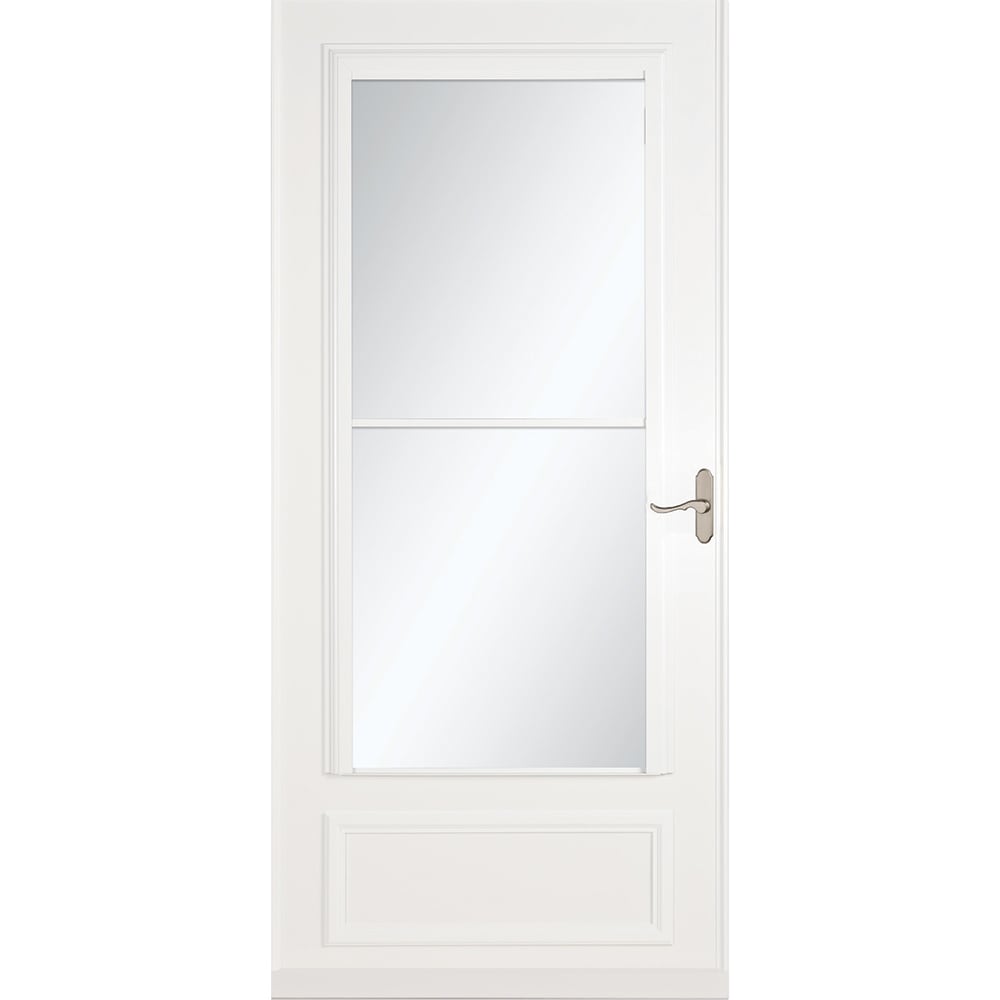The photograph features a white door with a sleek, modern design. The door has a pristine white frame and showcases two large, slightly mirrored glass windows positioned vertically, one above the other, accentuated by a delicate trim of several layers. Below these windows, there is a small, intricately molded rectangular panel etched into the wood. The right side of the door is fitted with a stylish lever handle made of burnished chrome, mounted on an oval base with rounded edges, perfectly aligned and facing left. The entire scene is set against a solid white background, highlighting the door's elegant simplicity, likely intended to serve as an advertisement display.